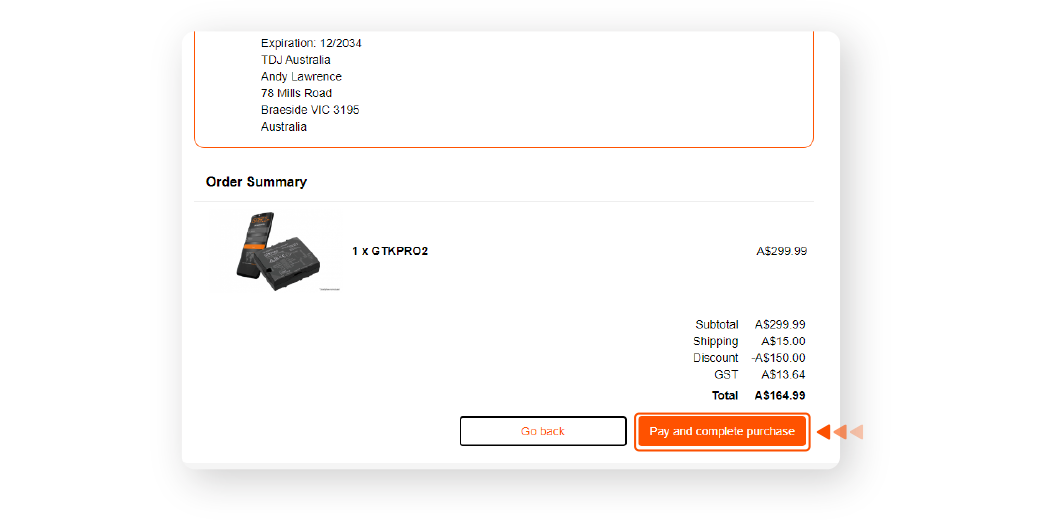In this image, there is a predominantly white background with elements featuring black, white, and orange colors. At the top of the screen, there is text that reads "Exploration 12-2034, TDJ Australia, Andy Lawrence, 78 Mills Road, Bradsco, VIC, 3195 Australia." Below this, a section labeled "Order Summary" is displayed. 

In the "Order Summary" section, two black rectangular or square devices, which appear to be either cell phones or batteries, are shown. Next to the image of these devices, the text "1XGTKPRO2" is displayed, followed by a price listed as "$299.99." The subtotal is also indicated as "$299.99."

Further down, additional costs are outlined: shipping is listed as "$15," a discount of "$150.00" is subtracted, and GST is noted as "$13.64." The total amount due is "$164.99."

At the bottom of the image, there are two buttons: a "Go Back" button and an orange "Pay & Complete Purchase" button with three orange arrows pointing towards it, emphasizing this option for finalizing the purchase.